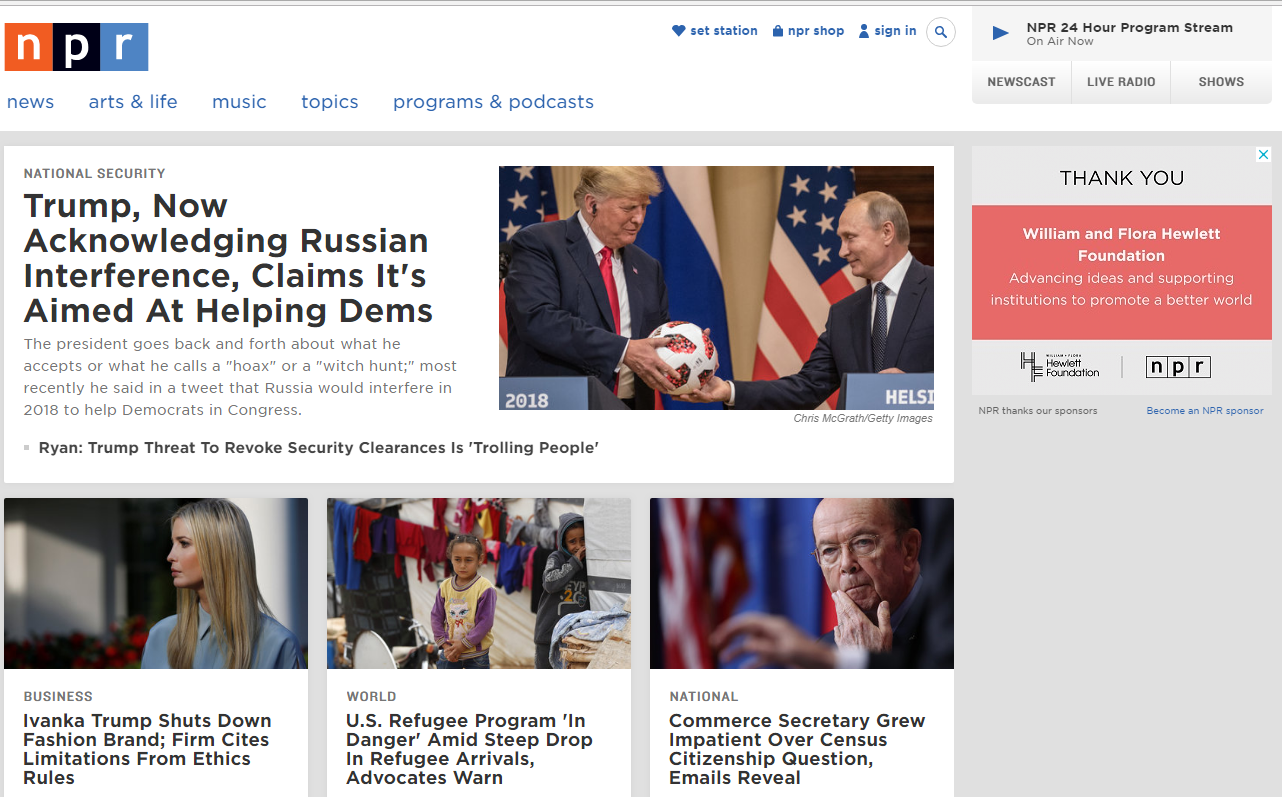**Caption for Screenshot of NPR Website:**

A detailed screenshot of the NPR website interface. At the top left corner, the iconic NPR logo is prominently displayed, featuring the letters "N," "P," and "R" in white, each enclosed in orange, black, and blue squares respectively. Next to the logo are options for setting a favorite station, accessing the NPR shop, and signing in. 

On the right side of the header, a gray vertical box provides links to the NPR 24-hour program stream, the newscast, and live radio shows. 

Directly beneath this menu, there is a banner extending gratitude with the text "Thank you" in a pinkish mango hue, acknowledging the William M. Flora Foundation and the Hewitt Foundation for their support in advancing ideas.

The website’s layout features a navigation bar on the left with categories such as news, art, life, music, and topics. Under the "National Security" heading, there is a highlighted article titled "Trump Now Acknowledging Russia Interference, Claims It's Aimed at Helping the Democrats."

Below the main article are three images with corresponding articles. The first image is of Ivana Trump, the second of a refugee, and the third related to a secretary for impatience, representing articles from the business, world, and national sections respectively.